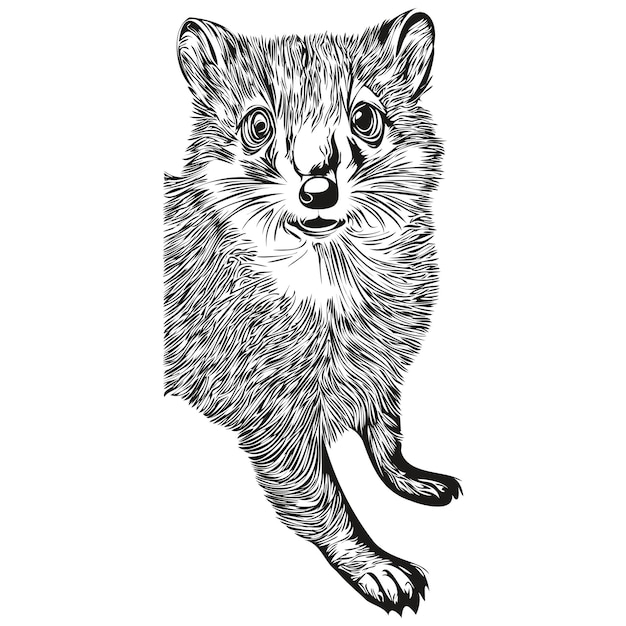This black and white sketch depicts the front portion of a small woodland animal, possibly a fox, dog, or squirrel. The drawing captures the animal's head, upper body, and two front paws, while the rest of its body is cut off. Rendered in what appears to be a black pen against a white background, the fur, eyes, and facial features are delineated with careful line work. The animal's face, which seems asymmetrical, features a little black nose, a small open mouth, and forward-facing eyes. Its rounded ears, detailed whiskers, and sharp claws add to the characteristics. The exact species of the animal is ambiguous due to its black and white depiction, but the detailed sketch provides a glimpse into the creature's enigmatic identity.